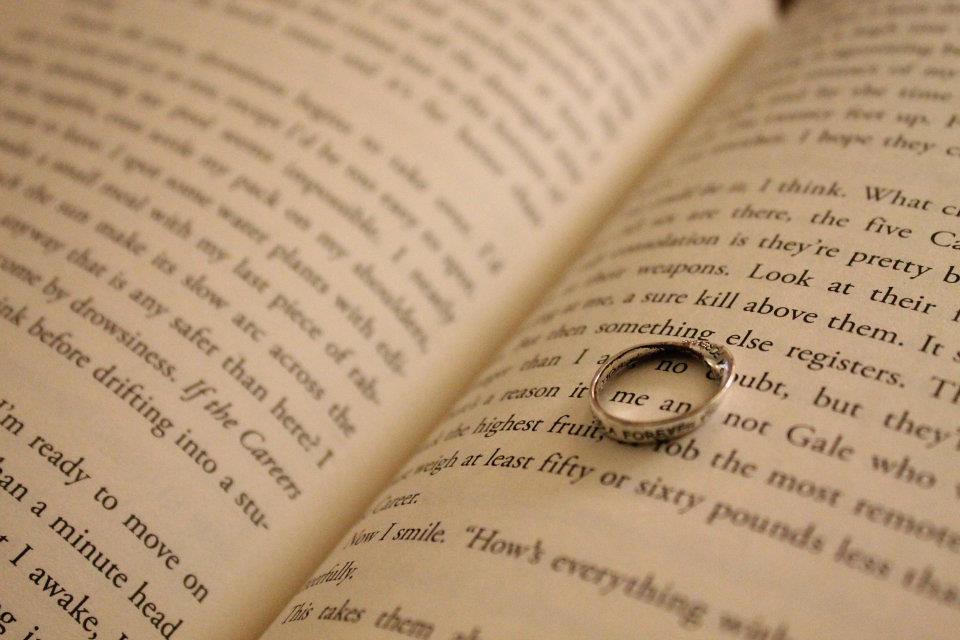The image captures a close-up of an open book, where the central crease is prominently visible, extending from the bottom left to the top right. The pages, an off-white color with black text, are partially blurred at the top, becoming clearer towards the bottom. On the bottom left corner, a legible text reads, "I'm ready to move on, then a minute ahead I awake," while the right page features clearer text near the center, stating, "look at there, they sure kill above them. When something else registers, then I am no doubt, but they reason it to me, and not Gail, who the highest fruit, robbed the most remote, weigh at least fifty or sixty pounds less than career. Now I smile, how's everything, successfully, this takes them." Placed on the right page, just below the middle of the image, is a silver ring engraved with the words "forever ingrained," facing the camera. This ring, possibly a wedding band, lies on the flatly opened book, emphasizing the connection between the everlasting inscription and the written words on the page.